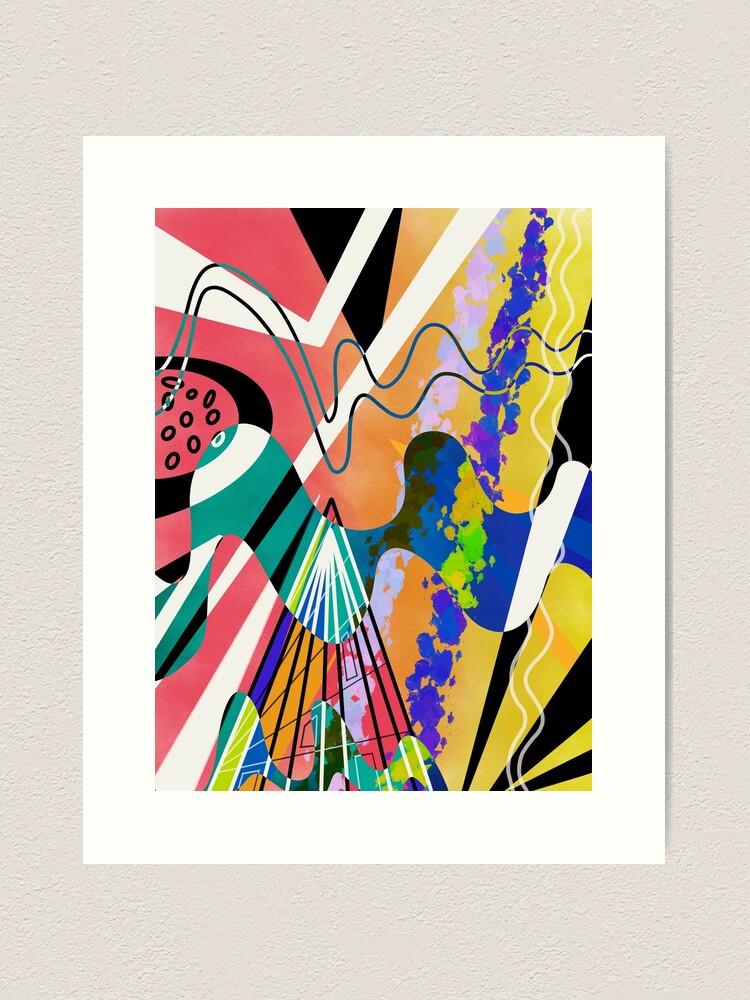This image showcases an abstract modern art painting, bordered by a thick white frame. Dominated by a vivid array of colors including shades of red, watermelon pink, orange, yellow, green, blue, teal, and black, the composition is a mesmerizing interplay of shapes and patterns. Swirling squiggly lines, resembling voice patterns, traverse horizontally across the canvas in colors such as teal and black. The background also features chevron-like white slashes and thick white vertical stripes that stretch from top to bottom. 

Near the top, there are contrasting black shapes, notably a black arrow towards the left and black slants peppered throughout. Meanwhile, a vibrant array of ovals and a large, multicolored squiggle—composed of teal, black, white, blue, lime green, and yellow—cuts through the center. The left side of the artwork predominantly displays warmer hues like watermelon pink and orange, transitioning to yellow on the right, with a blue and white splatter trail adding an unpredictable touch. Despite its lack of distinct structure, the dynamic flow of lines, colors, and forms creates a lively and compelling visual experience, making the painting a captivating piece of abstract artwork.